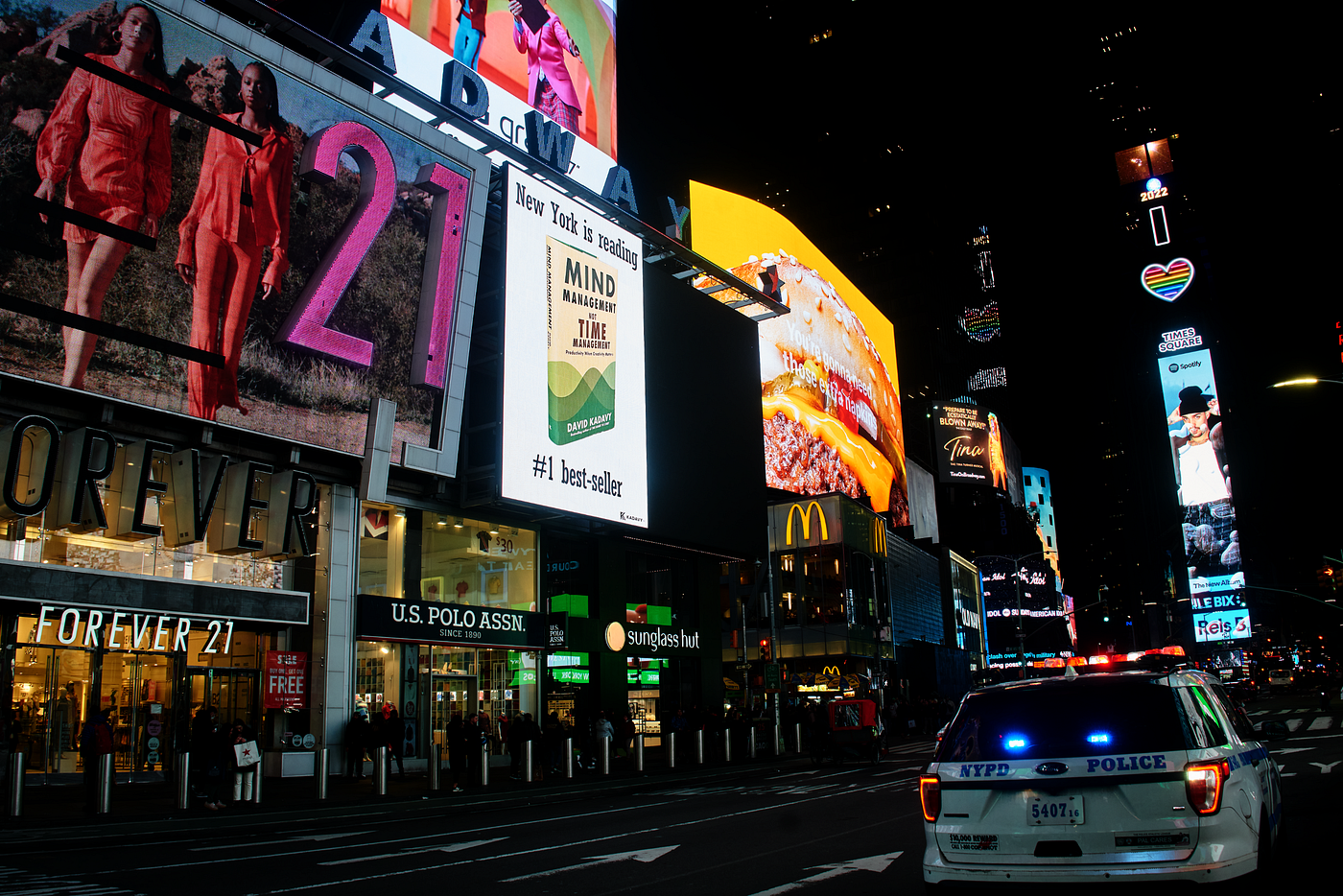The photo captures a bustling city street at night, likely in Manhattan, New York City. Dominating the bottom right corner is a white NYPD police vehicle with red flashing lights and its brake lights on, driving slightly away to the right. The street, lined with small white posts along the sidewalk, bends downwards and to the right, leading into a scene filled with tall, illuminated buildings.

To the left of the police car, several stores are visible including Forever 21, US Polo Assn., Sunglass Hut, and a McDonald's with its iconic logo. Above these stores, a series of bright billboards illuminate the night. One billboard displays two female models above the Forever 21 store, another showcases a book cover with "New York is reading" and "number one bestseller" captions, and a third advertises a hamburger above McDonald's. Further to the right is a tall vertical billboard featuring a man who appears to be of Hispanic descent, crowned by a heart with rainbow stripes.

In the top-right portion of the image, the outlines of more tall, illuminated buildings rise against the dark sky, enhancing the lively nighttime cityscape. The setting, with its mix of commercial signage and iconic urban elements, strongly suggests a location like Times Square.